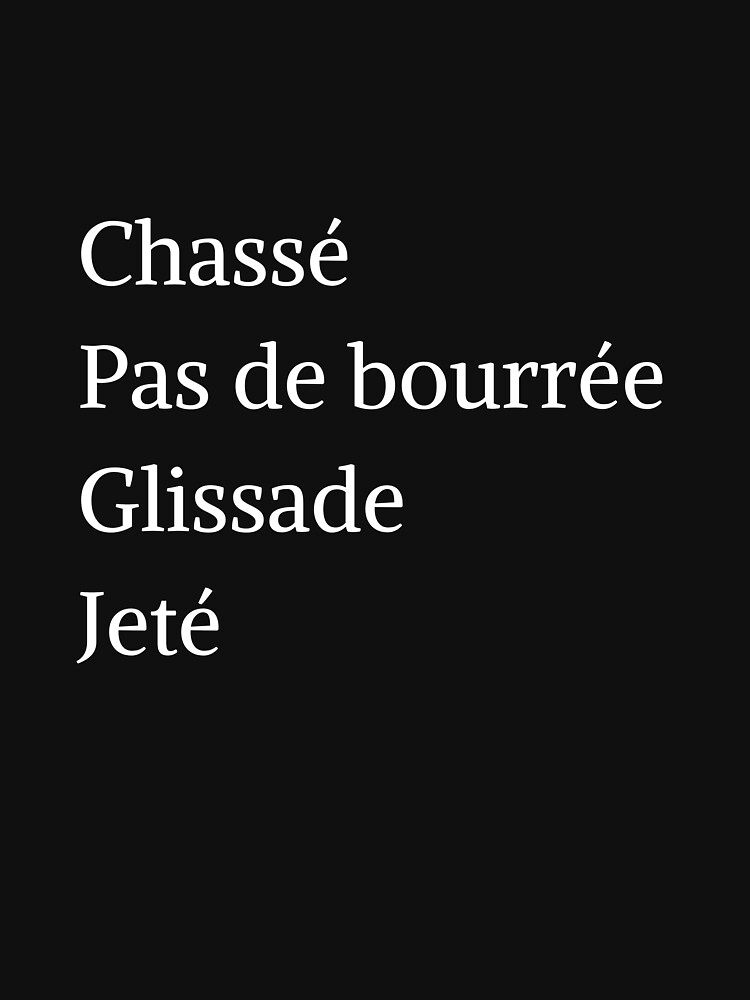The image features a simple, portrait layout with a deep black background and four lines of white text, all starting with capital letters. Positioned towards the left of the image, the text starts near the top and extends to the middle. The first line reads "Chassé," with the word spelled C-H-A-S-S-E, where the final "é" has an accent mark. The second line states "Pas de Bourrée," spelled P-A-S D-E B-O-U-R-R-E-E, with an accent over the second-to-last "é." The third line reads "Glissade," spelled G-L-I-S-S-A-D-E. The final line says "Jeté," spelled J-E-T-E, with an accent mark above the last "é." There are no other elements, colors, or people in the image, making the focus solely on the elegantly accented French dance terms in white text against a stark black backdrop.